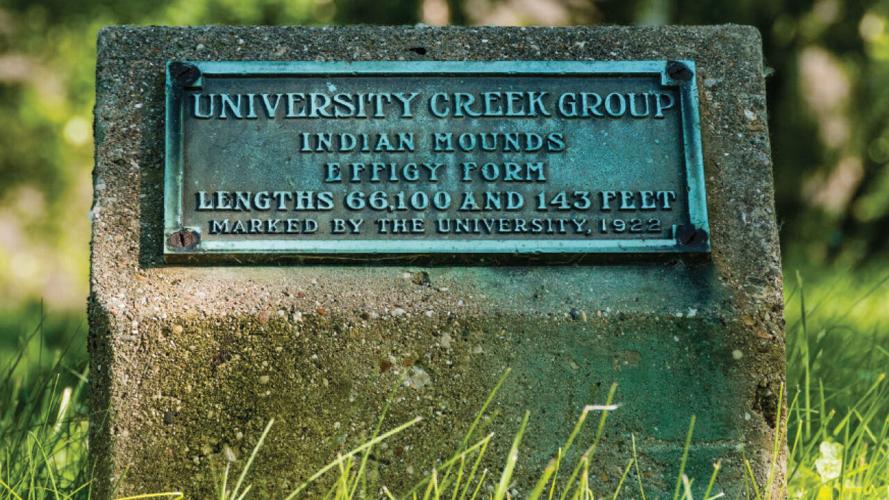This detailed photograph captures a weathered tombstone in a graveyard, prominently featured in sharp focus against a blurred, forested background. The ancient tombstone is constructed from crude stone, exhibiting significant wear and damage over the years, with a color palette of gray, brown, and green. Dominating the tombstone is an aged metal plaque, green with patina, inscribed with the details: "University Creek Group, Indian Mounds, Effigy Form. Lengths 66,143 feet. Marked by the University 1922." This scene is set in a grassy area, with blades of grass visible in the foreground. Sunlight filters through the surrounding trees, casting highlights and adding to the serene, historic atmosphere.